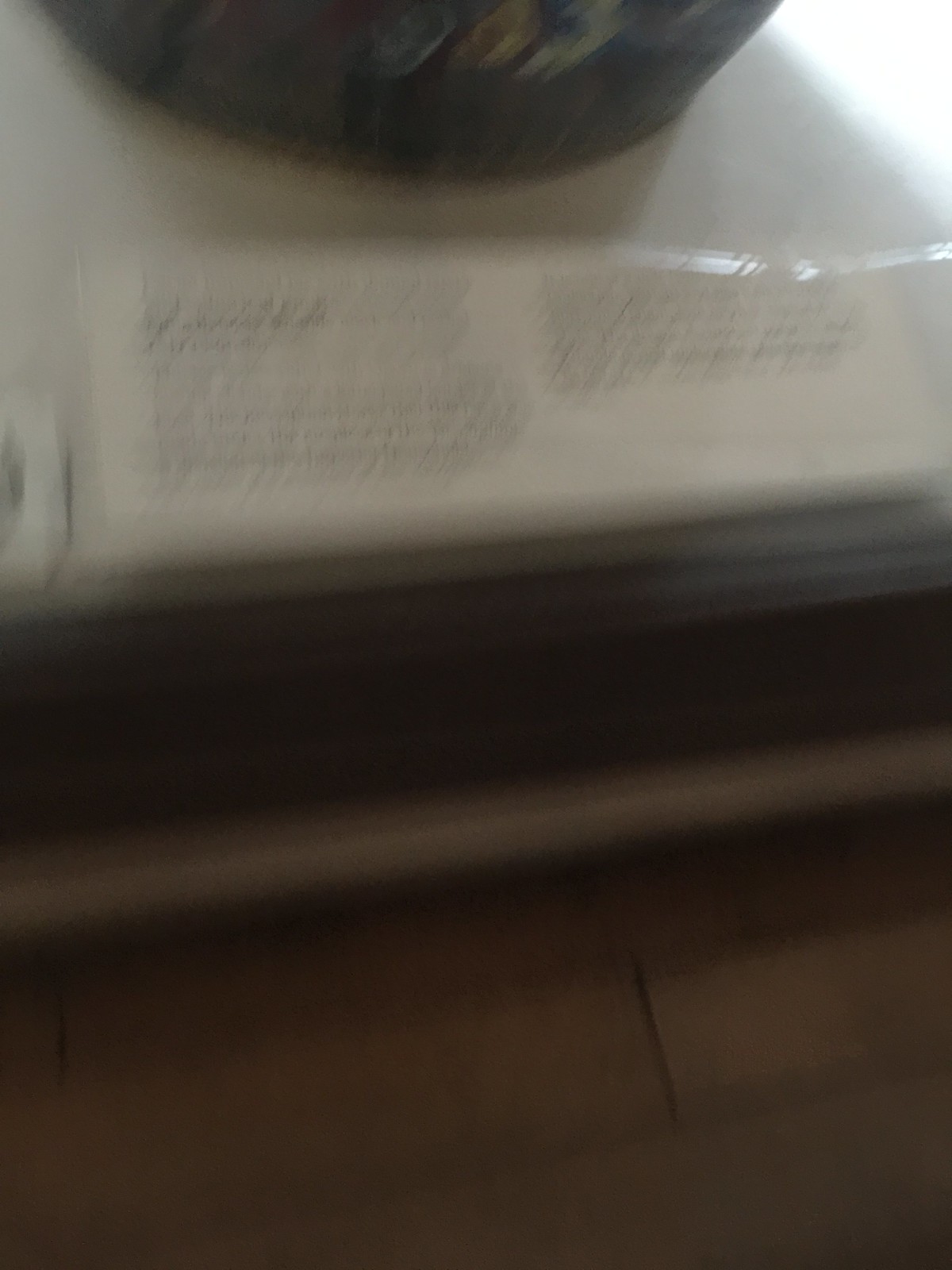A blurry, low-quality photo taken in a museum or similar exhibit space. The image captures the lower quarter of an unidentified object, possibly a bowl or vase, positioned on a white stand. The stand sits atop a dark brown base, contrasting with the lighter brown floor tiles visible at the bottom of the photo. In front of the object, a rectangular plaque with illegible black text is partially visible. The image's poor focus makes it difficult to discern finer details, such as the specific contents of the plaque or the exact nature of the object on display.